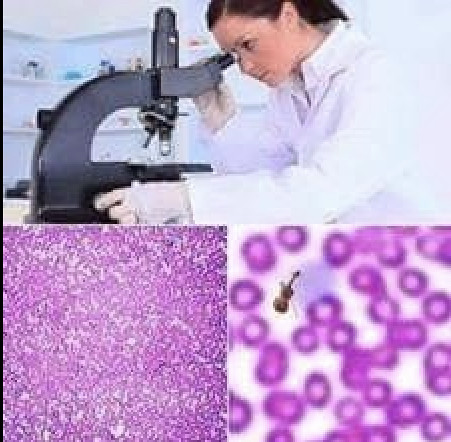In the image, the top section features a female scientist or lab technician with dark brown hair, dressed in a white lab coat and gloves, leaning in to observe something through a black microscope. She is in a well-organized laboratory setting with white shelving and various bottles in the background, indicating it could be a lab or pharmacy.

The bottom part of the image is divided into two sections. On the right side, there is a highly zoomed-in view of her observation, revealing colorful lavender-colored cells or microbes scattered across a white background, with what appears to be a tiny violin at the center, suggesting an element of humor. The left side shows a slightly less zoomed-in perspective, with these purple dots more spread out against the same white background.

Overall, the image combines scientific precision with a playful twist, depicting the dedicated work of a lab professional examining microscopic elements that whimsically include the world's smallest violin.